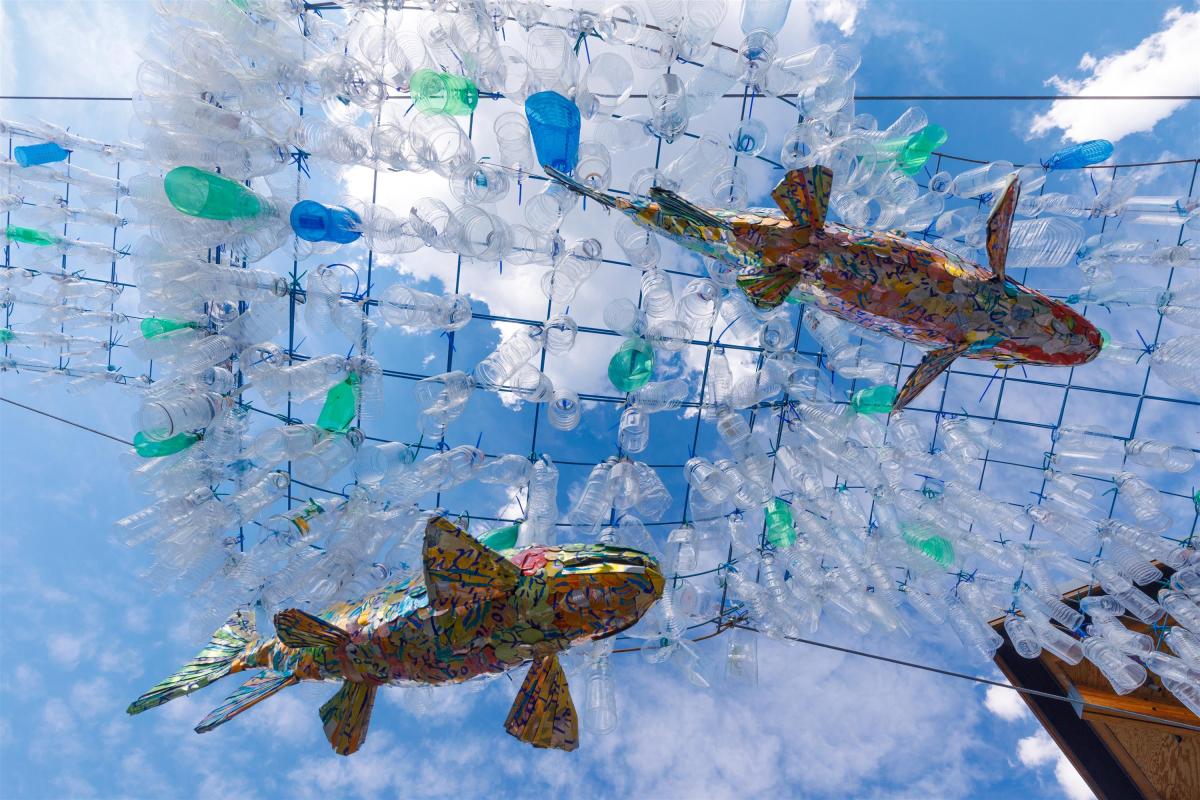A detailed painting captures two vibrant, multi-colored koi fish swimming beneath a black mesh net against a bright blue sky with scattered white clouds. The artwork is viewed from the underside, giving a unique perspective as if looking up from underwater. The fish are adorned with a spectrum of colors including yellows, blues, reds, greens, whites, and golds. One koi is positioned in the upper right, oriented to the right, while the other koi is in the lower left, also swimming to the right but angled slightly upwards. Their fins and tail are clearly visible, adding to the dynamic composition. The net in the background, composed of intersecting black lines forming square shapes, stretches across the scene, adding a layer of complexity and intrigue to the overall depiction.